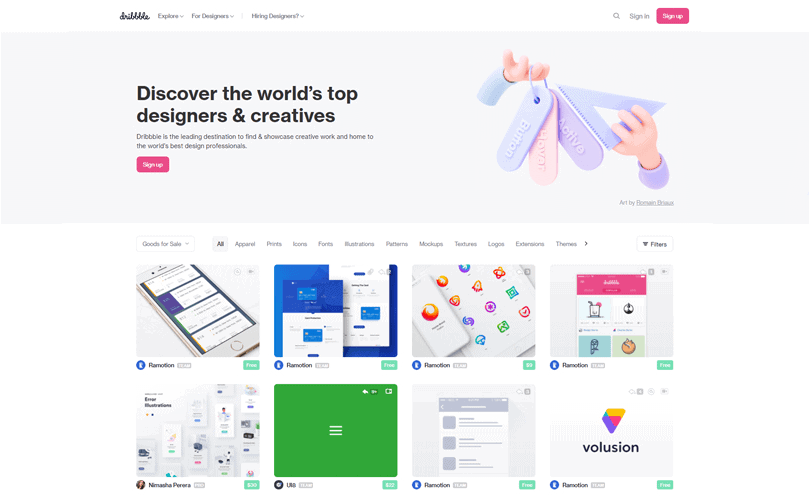This screenshot appears to be taken from the Dribbble website. In the upper left-hand corner, the word "Dribbble" is prominently displayed in bold, cursive lettering. To its right, there is a navigation menu that includes three items: "Explore," "Explore Designers," and "Hiring Designers," each with a drop-down option. 

In the upper right-hand corner, there are two buttons: a sign-in button and a red sign-up button. Below this header section is a prominent banner. Centered within this banner is the text, "Discover the World's Top Designers and Creatives," accompanied by a red sign-up button beneath it.

The right-hand side of the banner features an image of two hands, resembling clay animation figures, grasping various tools, including one that appears to be for drawing or cutting straight lines. Below this banner, there are two rows showcasing different items, each represented by an image, presumably illustrating the website’s various offerings.